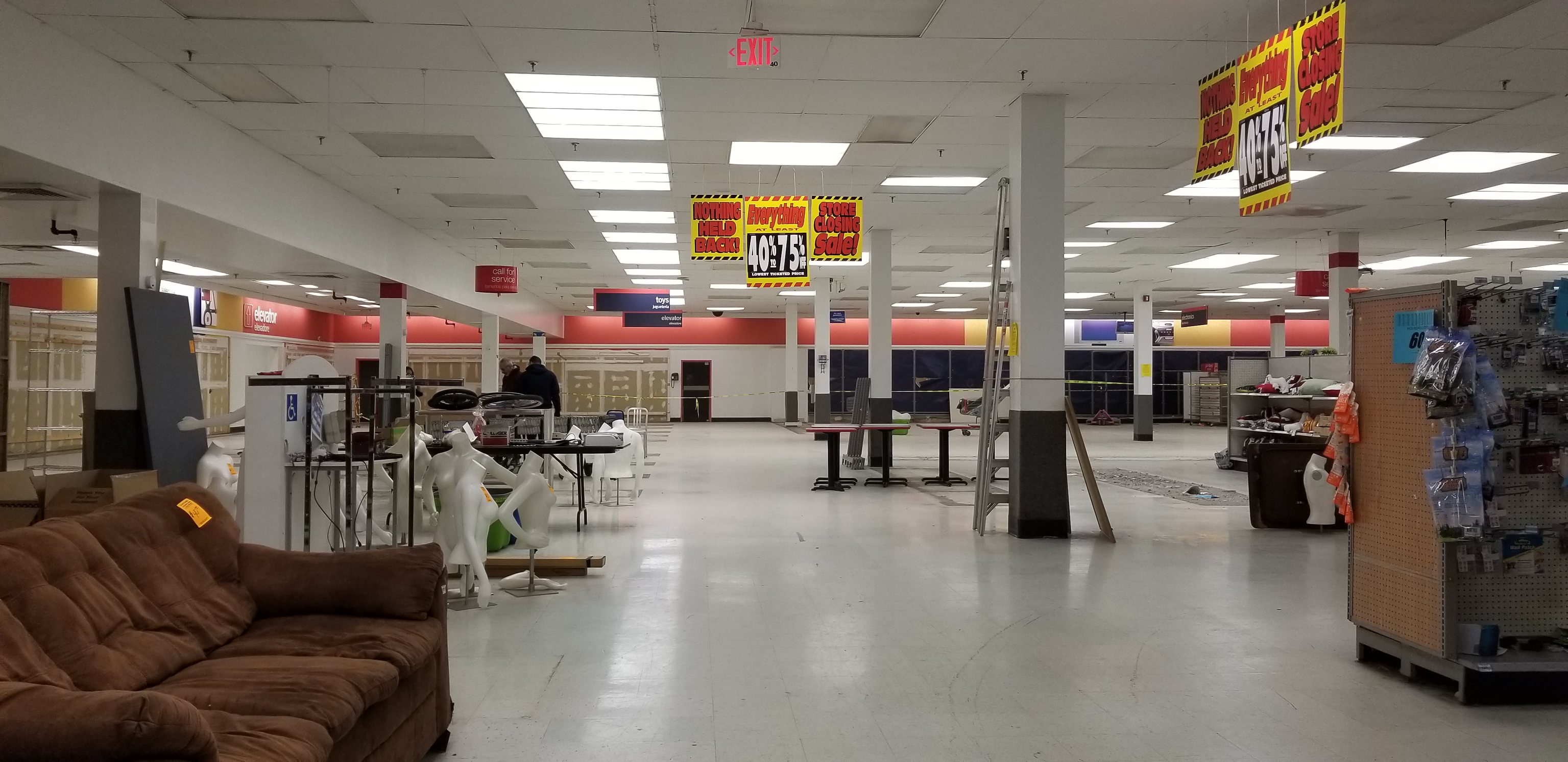This image captures a vast, almost cavernous commercial retail space that appears to be largely empty, possibly after a major sale. Prominent red and yellow signs, along with large black banners displaying "40" and "75," suggest significant discounts, though the finer details on the signs are not legible. The store's ambiance is dim, characteristic of an off-hours lighting schedule where only selective areas are illuminated. On the left side of the image, a brown couch with an orange tag, details unreadable, sits as one of the few discernible pieces of furniture. Nearby, a black door-like object, also featuring an unreadable orange tag, leans against one of the white pillars that dot the space. The ceiling is covered in white tiles typical of commercial interiors. Sporadic hints of red, yellow, and blue colors are visible throughout the store, adding sparse pops of color to an otherwise barren and abandoned shopping center.